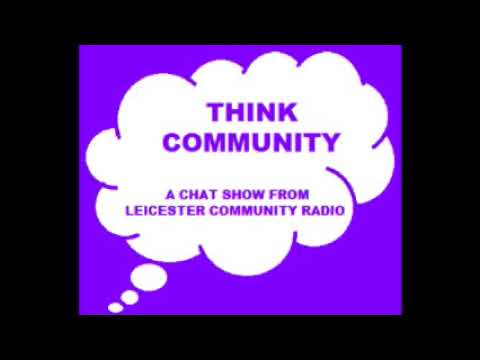The image depicts a pixelated advertisement featuring a central purple square icon with a surrounding black background, giving the impression of a framed picture. Dominating the center of the purple icon is a white, puffy thinking cloud with three smaller, white thought bubbles extending from its bottom left corner. In the upper half of the cloud, bold and darker purple text reads "THINK COMMUNITY" in all caps. Beneath this, in a smaller and slightly brighter purple font, the advertisement states, "A CHAT SHOW FROM LEICESTER COMMUNITY RADIO." The overall design is simple, employing only three colors: purple, white, and black.